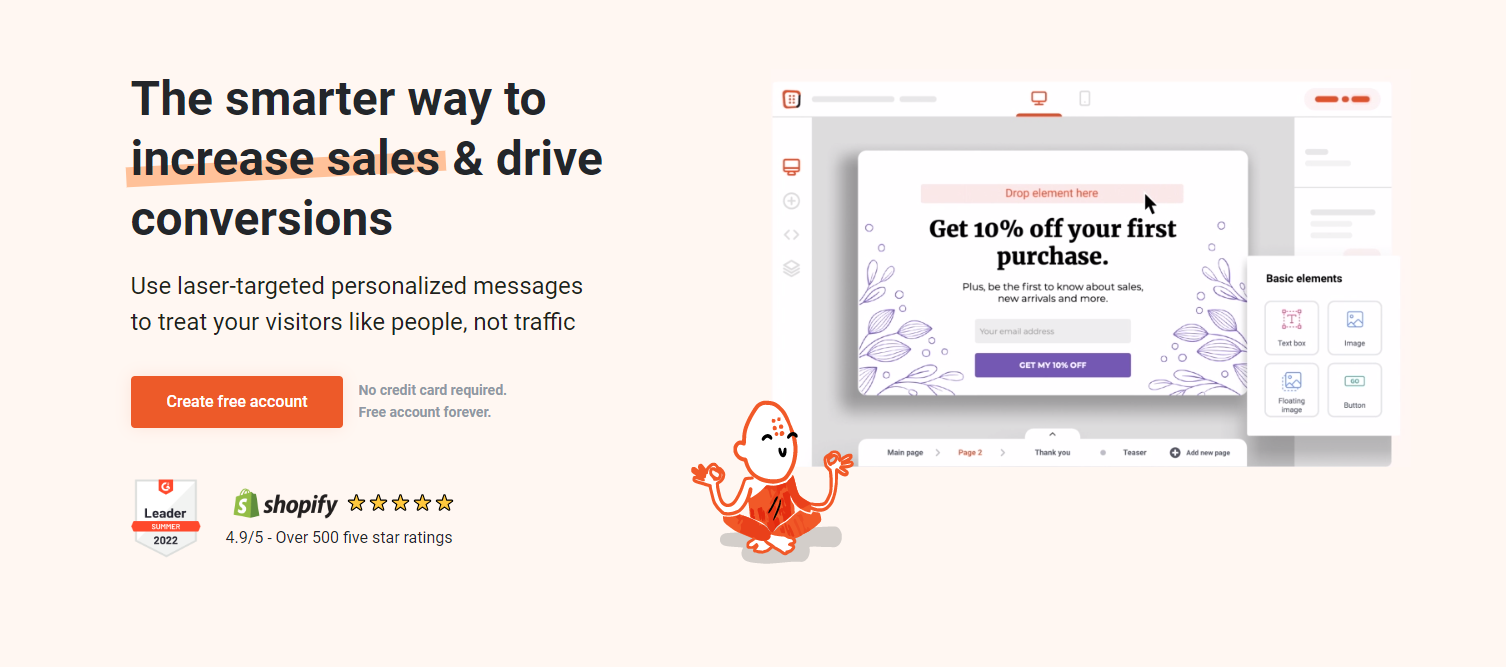The image showcases a platform designed to enhance sales and conversions by utilizing laser-targeted, personalized messages. The webpage is set against a light pink background. On the left side, bold text emphasizes, "The smarter way to increase sales and drive conversions. Use laser-targeted, personalized messages to treat your visitors like people, not traffic." Below this statement, an orange rectangle prominently features the call-to-action: "Create a free account. No credit card required. Free account forever." 

Further down, there's a certification label with "Leader Certified" adjacent to Shopify's logo, accompanied by five yellow stars, signifying a 4.9 out of 5 rating based on over 500 five-star reviews.

On the right side of the image, there is a screenshot demonstrating what the platform's interface looks like. Within this interface, a section invites users to "Drop element here" and promotes a 10% discount offer on the first purchase, along with early notifications about sales and new arrivals. This part includes a blank field for users to input their email addresses, and a purple rectangle with the prompt "Get my 10% off" in white text.

To the right of this central offer, there are a few white squares labeled, "Text Box," "Image," "Floating Image," and "Button," which likely represent customizable elements for user interaction. At the bottom of the screenshot, a rectangular drop-down menu displays navigation options labeled: "Main Page," "Page Two" (highlighted in red to indicate the current view), "Thank you," "Teaser," and "Add New Page." The image does not contain any additional text beyond these elements.